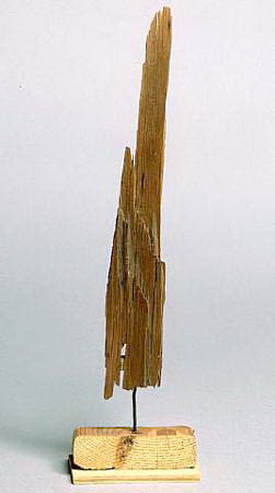The image showcases an abstract wood sculpture set against a neutral, gray background. The central feature is a long, narrow, and jagged piece of wood, resembling driftwood or balsa wood, which appears delicate and fibrous. This wooden piece extends vertically and is propped up by a tiny spike or wire that affixes it to a thin, rectangular block of plywood. Beneath this block is a thicker piece of flat wood, forming a stable base for the sculpture. The overall composition includes varied wood textures and colors, predominantly browns, beiges, and grays, contributing to its distinct, layered appearance.